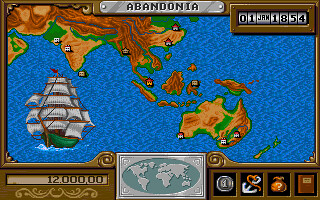This image depicts a small, rectangular screenshot of a retro, pixelated video game with a ship theme. The game screen is framed by a thin brown border at the top and a more prominent border around the sides. Centered at the top, a metallic silver banner displays the word "Abandonia" in black letters. In the top right corner, a date indicator shows "01 January 1854," likely reflecting the game's progression.

The primary play area features a sea dotted with islands and landmasses. Dominating the scene is a large, old-fashioned ship with prominent white sails and a green hull. 

At the bottom center of the image, a substantial silver rectangle contains a map of the world. The map is rendered with a blue ocean background and silver continents. To the left of this map display, another large rectangle indicates the in-game currency, with a current value of 12,000. On the right side, four smaller icons are positioned vertically, each representing different game elements: an anchor, a money bag, a book, and a silver coin.

This detailed and nostalgic screenshot captures the essence of vintage video gaming with its intricate design and clear visual storytelling.